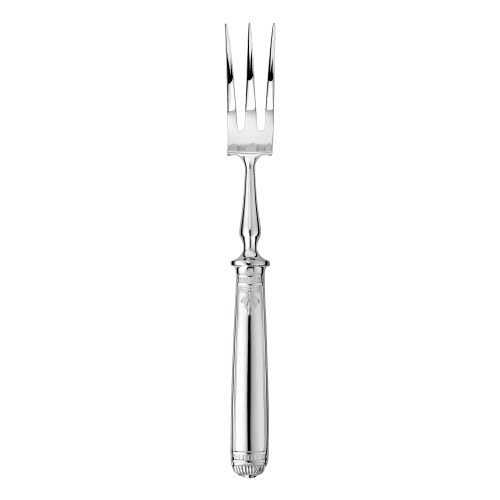The photograph prominently features a premium-quality, silver-plated dessert fork positioned upright against a plain white background. The fork, with its shiny and reflective surface, has three sharp, pointed tines that exhibit a hint of blackish shading near their base. The handle is thick, round, and cylindrical, adorned with intricate engravings and indentations that create a decorative border both at the top and bottom. The fork's design is intricate, with detailed carvings extending to the very bottom of the handle. The utensil exudes a sense of elegance and craftsmanship, characteristic of high-end silverware. Additionally, there is writing at the base of the fork, contributing to its distinct and ornate appearance.